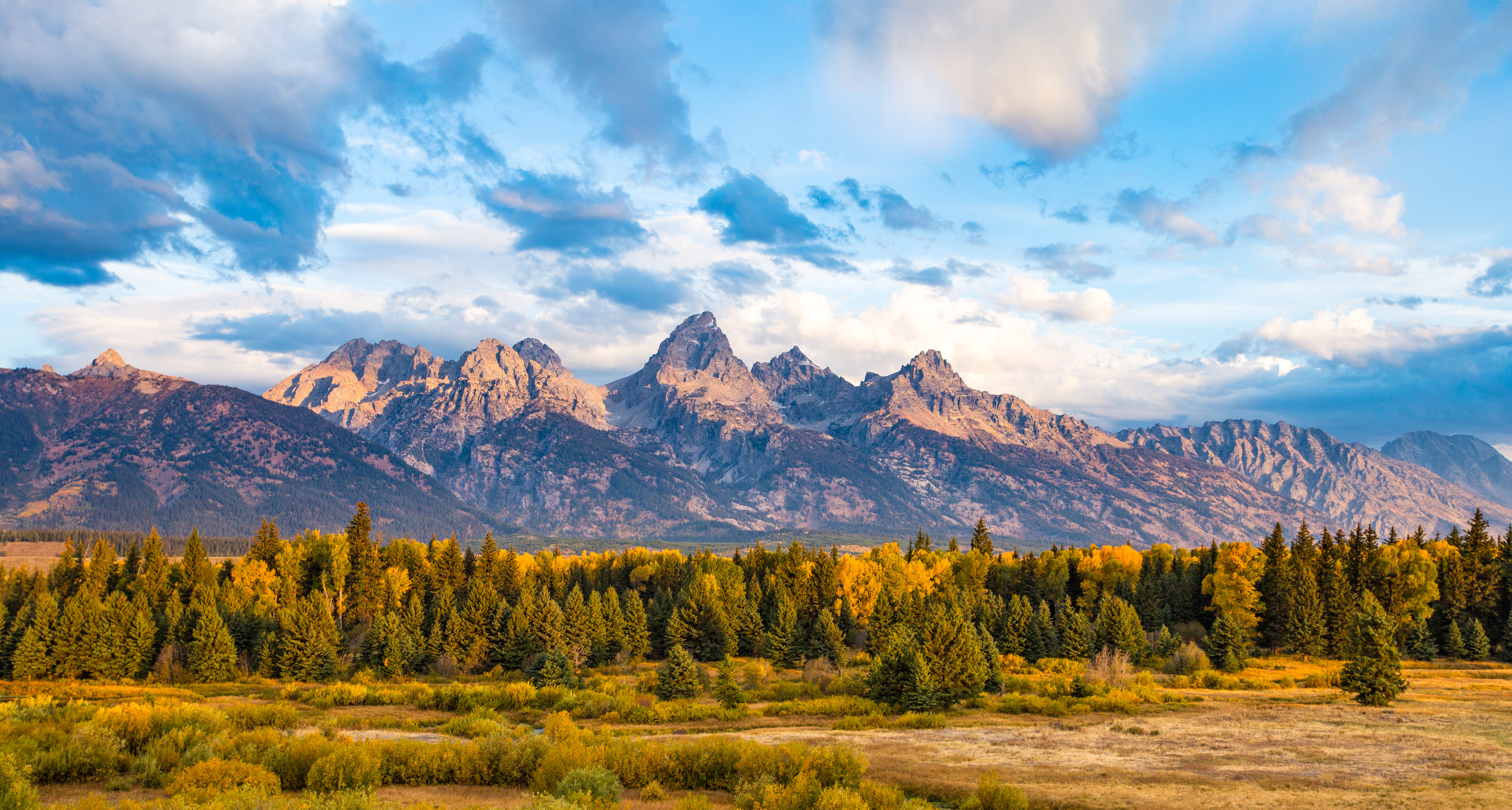The photograph is a full-color, horizontally rectangular outdoor nature shot taken in daylight. The top half of the image features a clear blue sky with white clouds, some tinged with a darker hue. Below the sky stretches a mountain range with brown and grayish rock, illuminated by sunlight and devoid of snow or substantial vegetation. Beneath the mountains is a dense row of pine trees, creating a green, forested layer. In the bottom right corner lies an open field with patches of greenery and brown soil, while the center lower left area contains green bushes or smaller plants. The scene captures the essence of a scenic outdoor location bathed in natural daylight.